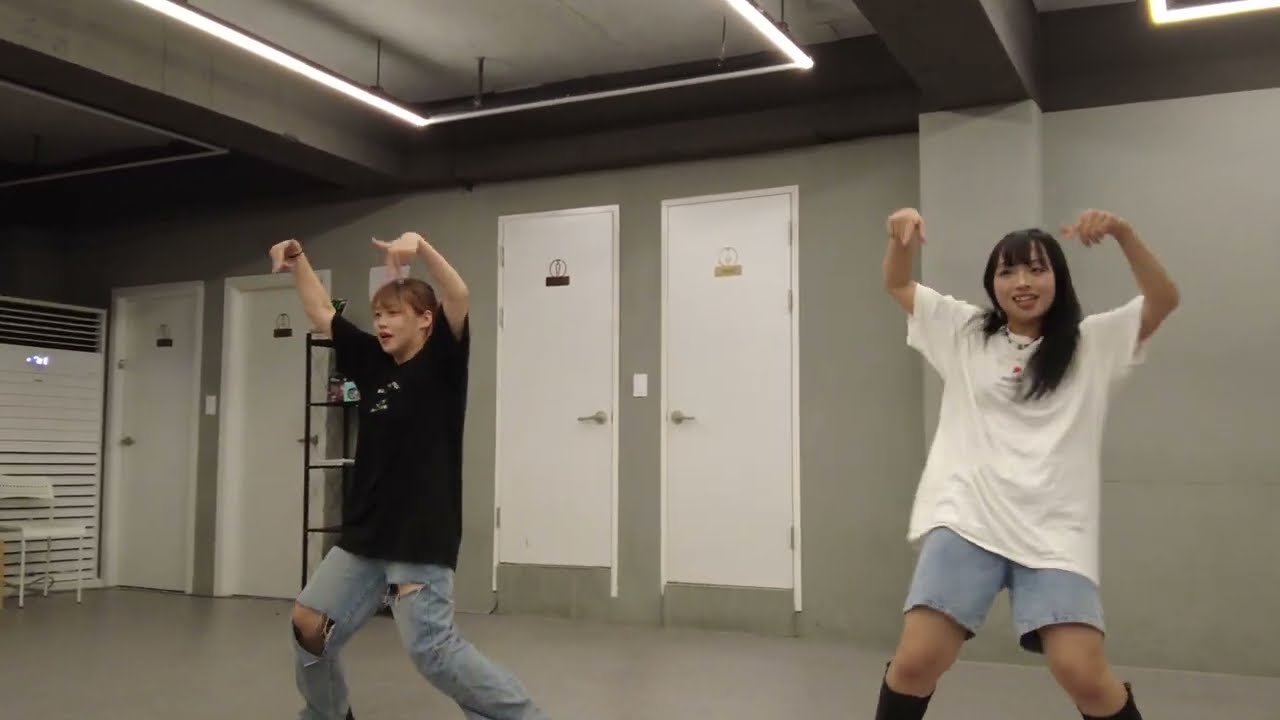The image features two Asian girls engaged in what appears to be a dance routine in an indoor studio or gymnasium. Both girls have their knees bent and arms raised with fingers pointed downward, suggestive of a hip-hop dance or similar style. The girl on the left is wearing a short-sleeved black t-shirt, light blue ripped jeans, and has dark brown, possibly dyed, hair. She is facing slightly to the left and forward. The girl on the right is dressed in a short-sleeved white polo shirt, light blue jean shorts, and black boots or high socks. Her long black hair falls to around her chest. Both girls are smiling as they dance on a smooth gray concrete floor. The backdrop features a gray wall with a set of two white doors in the center and potentially two more elevated doors on the left that lack doorsteps, creating an unusual visual. The ceiling has industrial features with rectangular white light fixtures, contributing to the stark, monochromatic aesthetics of the studio environment.